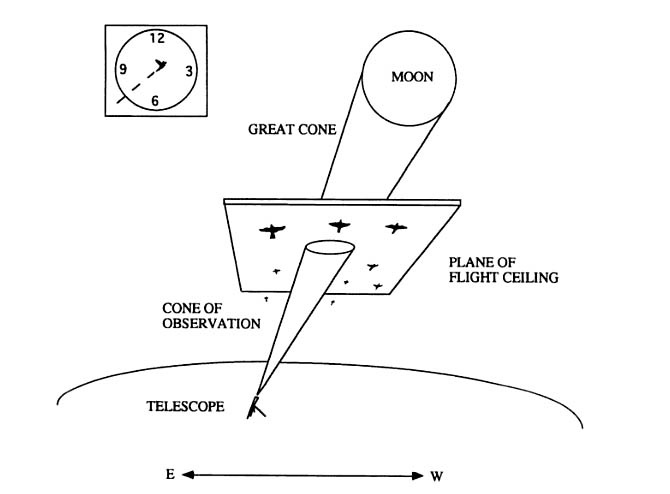The image is a simplified digital illustration, likely created in a program like Microsoft Paint, depicting the workings of a telescope. At the bottom, there's a small, rudimentary, sketched depiction of a telescope, standing on a tripod, labeled "telescope." Below this label is a double-sided arrow with 'E' on the left and 'W' on the right, with a small half-circle above it cradling the telescope. 

Emanating from the telescope is a cone labeled "cone of observation," which extends upward through a rectangular plane labeled "plane of flight ceiling." This plane features three rows of sketched birds in formation. Continuing upward, the cone widens and is labeled "great cone," culminating at a small, simplistic depiction of the moon. 

In addition, the top left corner of the image features a clock, with its long hand pointing around 8, though the shorter hand appears absent. The entire illustration is rendered in black and white, with all elements appearing as simplistic line drawings.